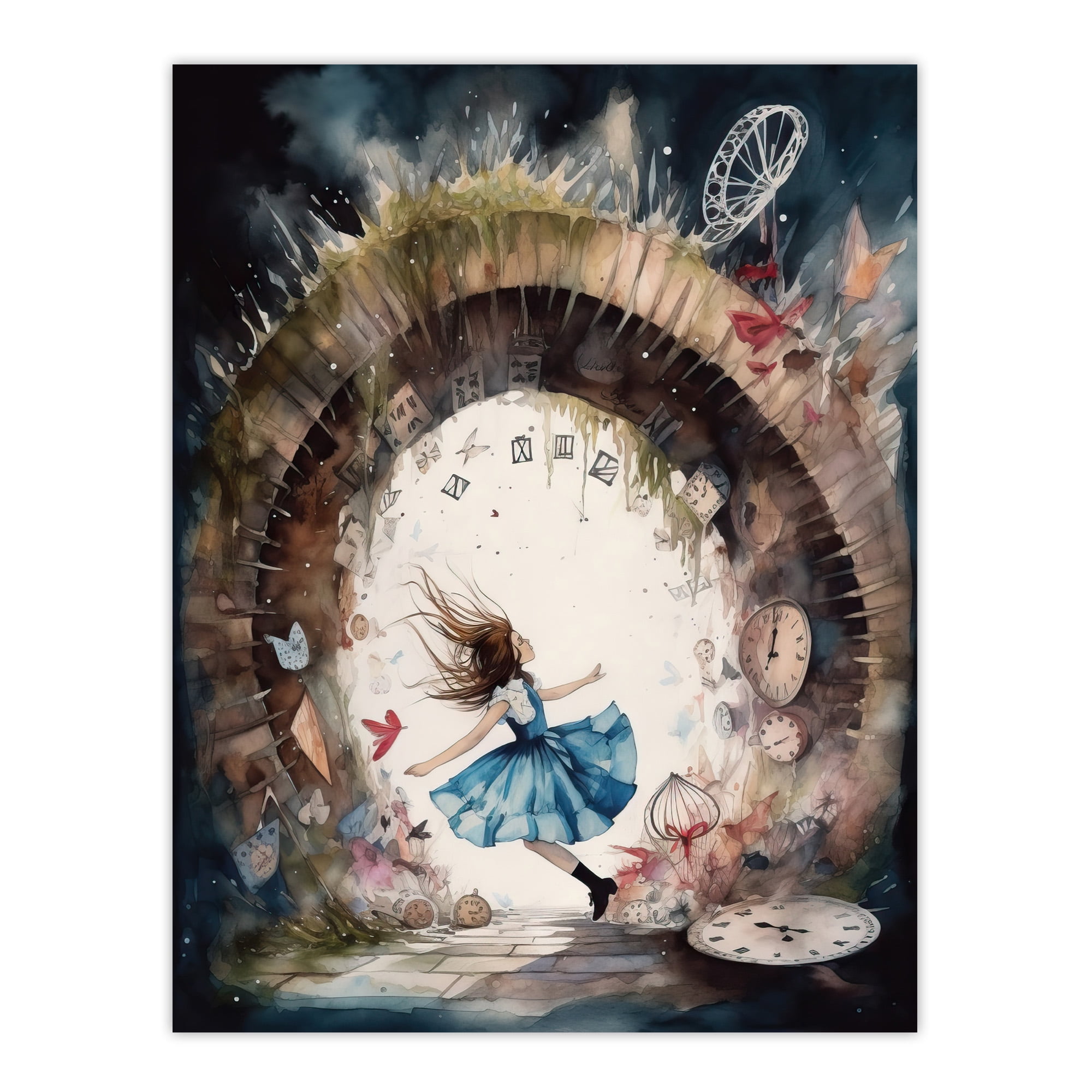This is a highly detailed watercolor painting depicting a scene evocative of Alice in Wonderland. At its center, Alice is portrayed wearing a blue dress with a white top, resembling a pinafore. Her brown hair is blown to the left, and she has an unusual feature of two left hands, with her left hand pointing behind her on the right side of her body. She appears to be emerging from or heading towards a stone archway that symbolizes a portal.

Surrounding Alice are a variety of objects, including wall clocks, trippy-looking alarm clocks, playing cards, papers, flowers, butterflies, and cute ribbons. The colors in the painting are vibrant and varied, with shades of blue, brown, red, peach, gray, and white contributing to the dreamlike atmosphere. The absence of text allows the viewer to fully immerse themselves in the whimsical and surreal elements depicted in the scene.